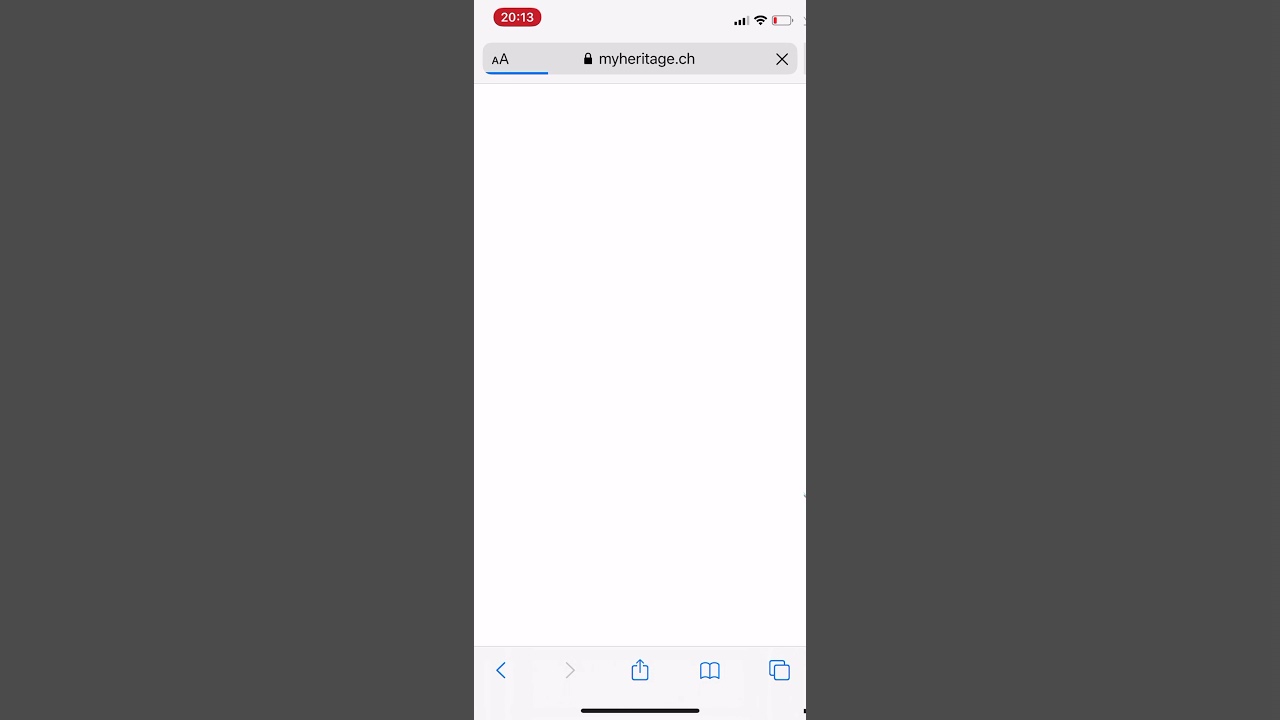This image is a detailed screenshot of a mobile phone display, showcasing an interface in a partially loaded state. The entire background features a large, dark gray rectangular box on the left side and a similarly large gray box on the right side, both larger than the actual screenshot itself, indicating perhaps an overlay or annotation.

At the very top left corner, there is a small, red oval shape displaying the numbers "20:13". Adjacent to this red oval are icons representing data, Wi-Fi connection, and battery life. The battery icon appears almost empty, distinguished by a narrow red bar indicating low charge.

Below this status bar, there's a search bar. On the left side of this bar, small 'A' and large 'A' icons are displayed, likely for text size adjustment. A blue line runs beneath these icons. To the right within the search bar is a lock icon labeled "myheritage.ch", suggesting this is the URL currently being accessed. On the far right inside the search bar, there is an 'X' icon.

The majority of the screen remains blank, appearing as a white page likely caught in the process of loading.

At the bottom of the screenshot, there is a navigation toolbar containing multiple icons. From left to right, these icons include two arrows (possibly for navigation), a box with an arrow pointing up (commonly representing a share function), something resembling an open book (perhaps for bookmarks or reading mode), and two overlapping squares. 

Overall, the screenshot provides a glimpse of a mobile web browsing session that has been disrupted or is incomplete.